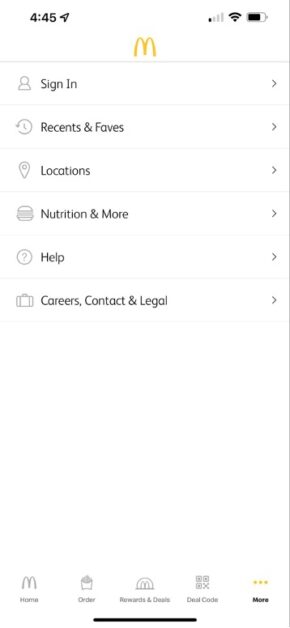This is a detailed screenshot from a cell phone displaying the McDonald's mobile application interface. At the top, the status bar shows the time as 4:45, along with the signal strength bars, Wi-Fi icon, and battery indicator on the right side. Dominating the center of the screen is the iconic McDonald's golden arches logo, without any accompanying text. Below the logo, various navigation icons are arranged in a list format:

- A person icon labeled "Sign In"
- A clock face icon with the label "Recents and Faves"
- A location pin icon marked "Locations"
- A hamburger icon reading "Nutrition and More"
- A question mark icon for "Help"
- A briefcase icon labeled "Careers, Contact, and Legal"

Each of these options has a right-pointing arrow indicating further selections are available.

At the bottom of the screen, there is a navigation bar with five icons:
- The golden arches labeled "Home"
- A French fries icon labeled "Order"
- An "M" inside a dome marked "Rewards & Deals"
- A QR code icon labeled "Deal Code"
- Three horizontal golden circles labeled "More"

The screen contains no photographic elements or images of animals, focusing solely on the interface and navigation options of the McDonald’s app.